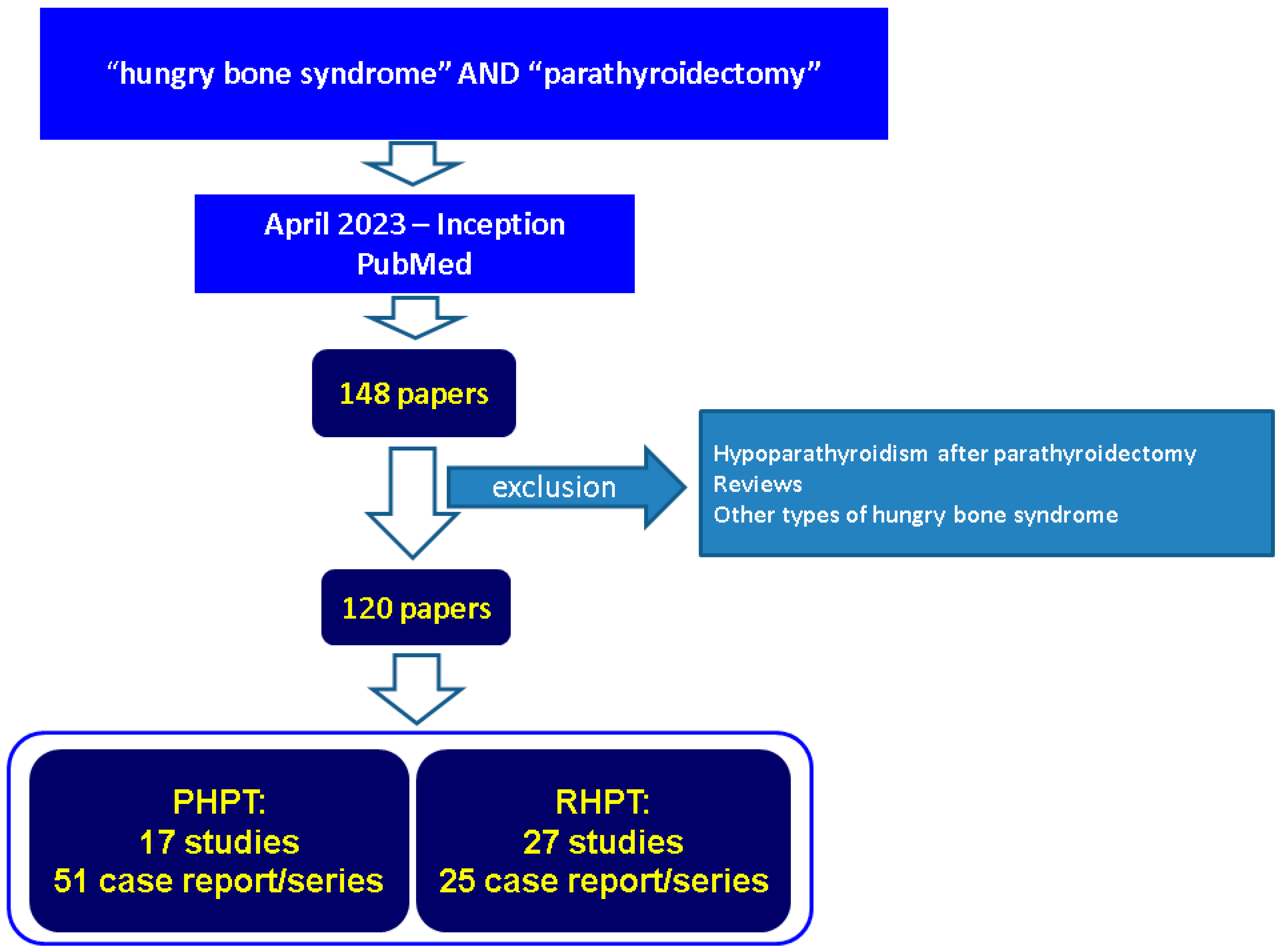The image displays a detailed flowchart diagram on a white background. At the top is a blue bar with white letters that read "Hungry Bone Syndrome and Parathyroidectomy." A downward arrow from this bar leads to another blue section labeled "April 2023 - Inception PubMed." Subsequent arrows point downwards to two more sections: one stating "148 papers" in dark blue with yellow letters and another saying "120 papers" also in dark blue with yellow letters. A larger rectangle at the bottom is divided into two sections. On the left, in a dark blue bar with yellow letters, it says "PHPT - 17 studies, 51 case report/series," while the right section, also in dark blue with yellow letters, reads "RHPT - 27 studies, 25 case report/series." A horizontal green arrow labeled "exclusion" leads to another section stating "Hypoparathyroidism after Parathyroidectomy reveals other types of Hungry Bone Syndrome" in light blue with white letters.